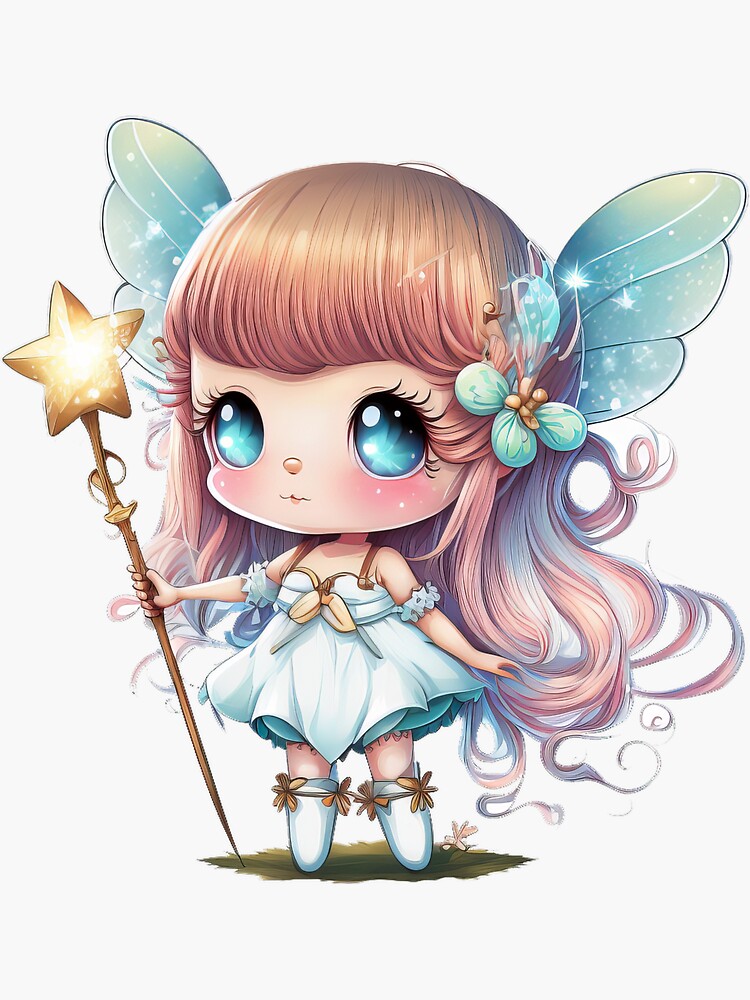The image showcases a detailed drawing of a young fairy-like girl with quite a large head compared to her body, accentuating her youth. She has long, wavy, light brown hair with bangs, adorned with a decorative headpiece resembling a twig with turquoise flowers. Her large blue eyes are striking, with little black accents around the blue, and her mouth is a small, closed line. She sports a light blue or turquoise dress with brown leather straps around her shoulders. Her delicate, fairy wings behind her are a light turquoise or blue-green color, matching various subtle hues in her attire. In one hand, she holds a stick or wand made of brown material, crowned with a glowing golden star. Her legs are adorned with white socks, and a sliver of green ground is visible beneath her feet. The background of the image is light gray or white, providing a clear and well-lit setting that highlights the enchanting elements of her fairy-like appearance.